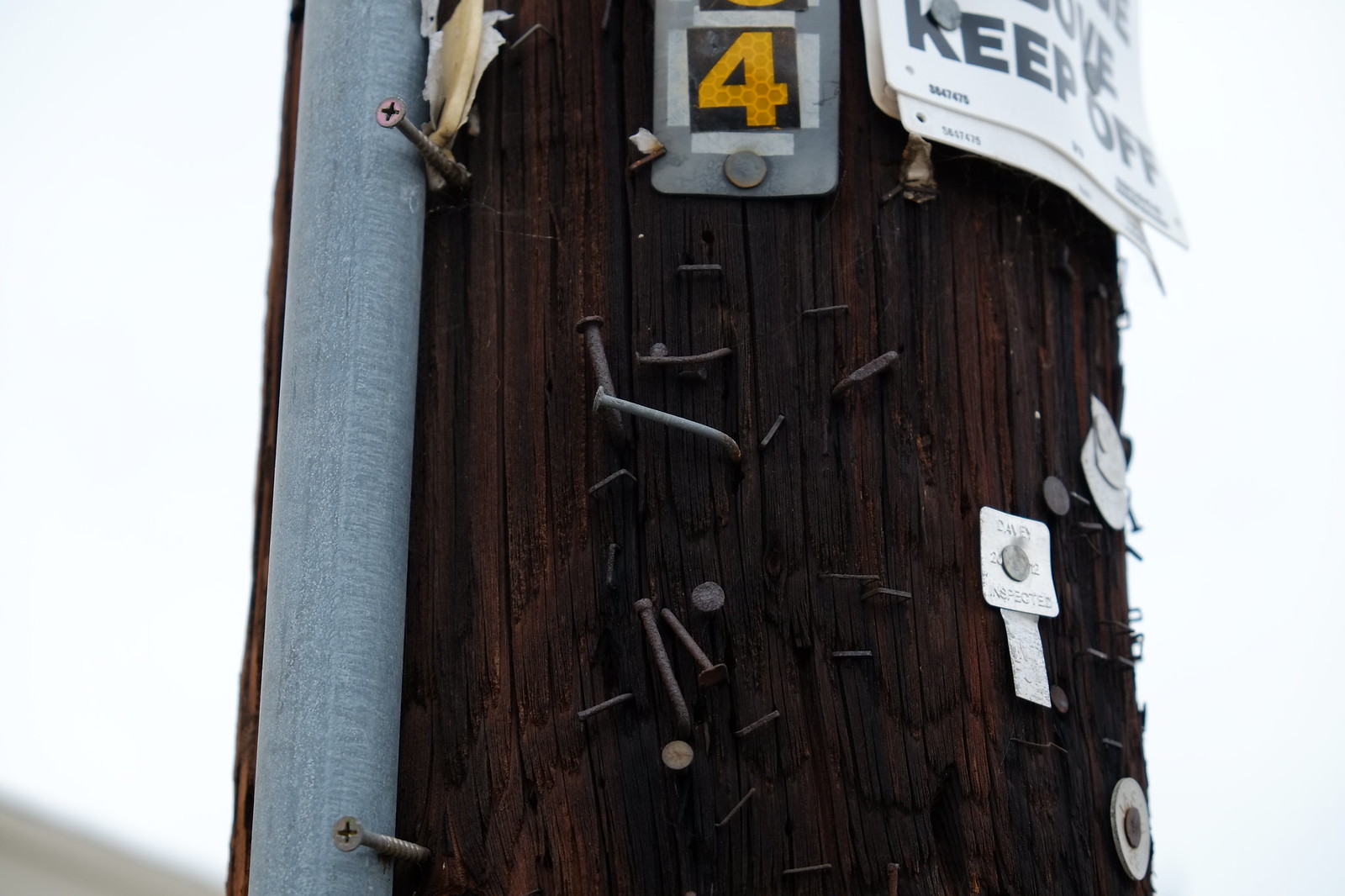The photograph captures an extremely detailed close-up of a weather-beaten telephone pole, darkly stained with black tar-like weatherproofing. The pole's surface is marked by the passage of time, evidenced by numerous old, rusted, and bent nails along with a myriad of staples. The wood itself appears dry and split in places, adding to its rustic, aged appearance. Along the pole runs a light gray or silver vertical conduit, possibly for wires, which is partly secured by screws.

A notable feature in the image is a partially visible white sign with the bold, capitalized command "KEEP OFF," suggesting various messages have been posted here over time. Near this sign, there is a galvanized metal strip affixed to the pole, displaying a bright orange number "4" bordered in black, likely reflective for visibility. The number is more permanently attached using silver tacks. Some Phillips head screws and remnants of previous postings, including fragments of paper, plastic, and other materials, are scattered across the pole, hinting at its long history as a community bulletin board. The pole is enveloped in a subtle ambient light, highlighting the textures and the remnants of countless flyers and posters that once decorated it.